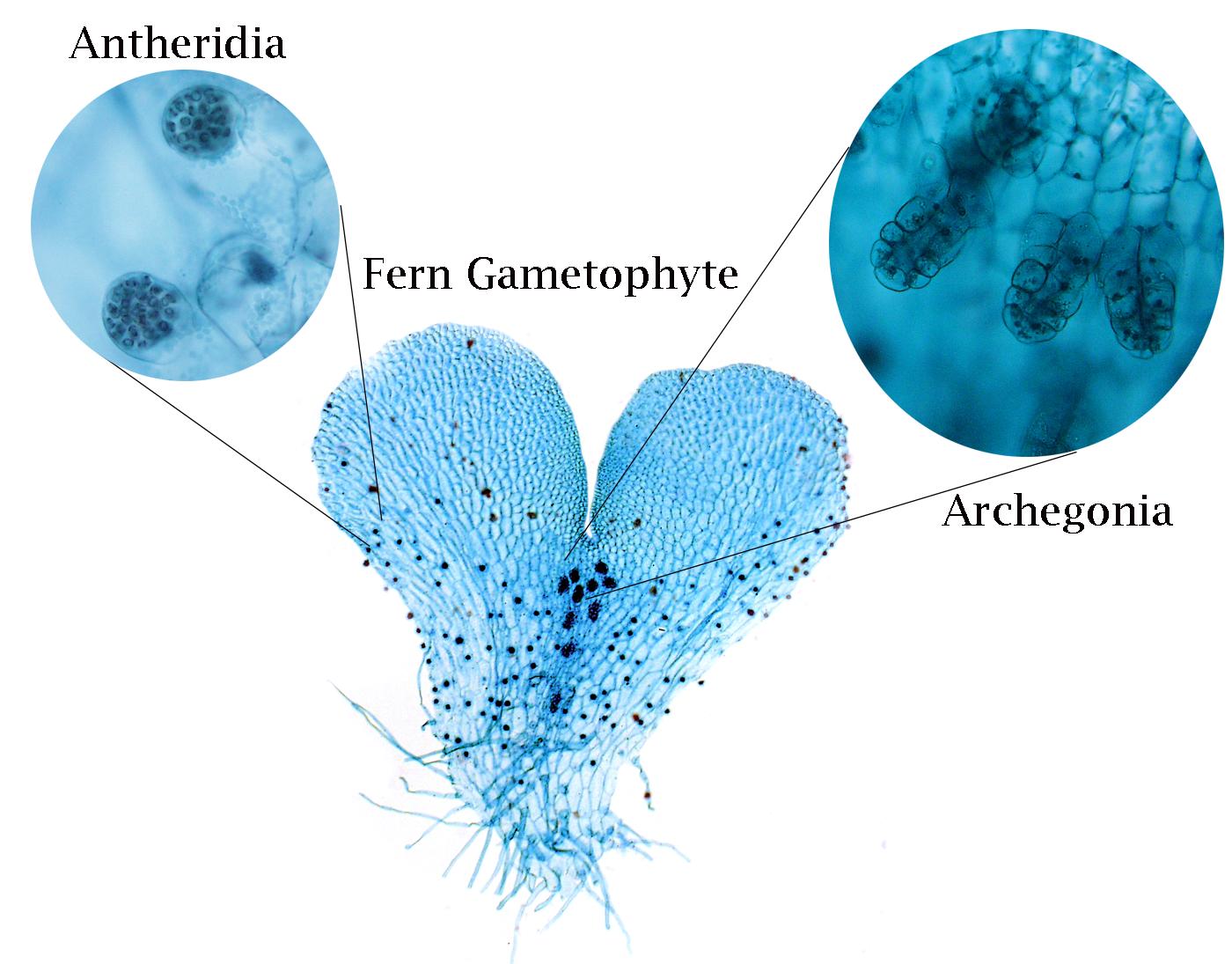The scientific illustration prominently features a central, heart-shaped fern gametophyte which is light blue with intricate lines running through it, converging at the bottom into protrusions. This fern gametophyte, with its conical and somewhat upside-down appearance, is labeled above in bold black letters. Small black dots are scattered throughout the structure. On the left side, a zoomed-in circular magnification labeled "Antheridia" displays two smaller black circles within a light blue and white background, illustrating finer cellular details. To the right, another magnified view is shown, a darker blue circular section labeled "Archegonia," which has a honeycomb-like texture at the top and three finger-like projections containing additional black dots. Black lines connect these magnified sections to their corresponding areas on the fern gametophyte, providing a comprehensive, detailed view of the cellular structures involved in this botanical diagram.